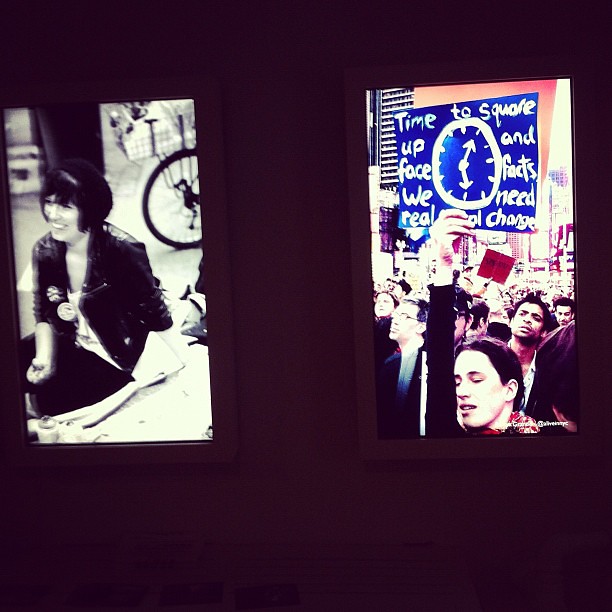The image features two framed photographs against a deep purple background. The photograph on the left is a black-and-white image of a woman sitting on the ground, facing left with a slight smile on her face. She is wearing a black jacket and appears to be outdoors, evidenced by a bicycle with a basket visible near her. The image is somewhat out of focus and tilted slightly to the left. The photograph on the right is in color and depicts a crowded demonstration or protest. Among the crowd, a prominent blue sign with white writing stands out, reading, "Time to square up and face facts. We need real change," with a clock showing the time around ten after six. Both photographs appear to be meticulously cut out and arranged on the dark purple background.